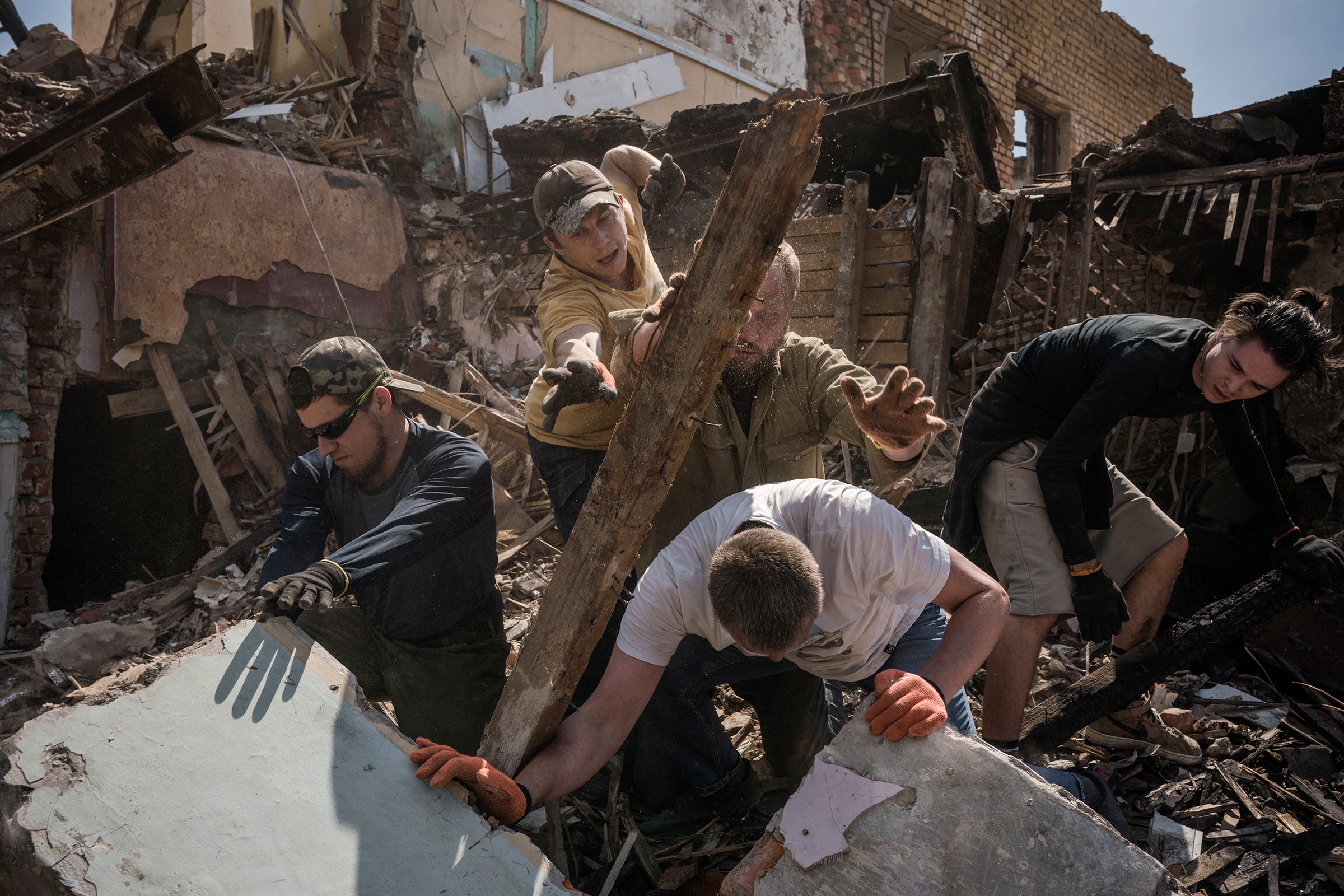The image captures the scene of a partially collapsed house, surrounded by debris and rubble, possibly the aftermath of a natural disaster or a controlled demolition. Six men, all wearing gloves—some black, some reddish-orange, and others grayish-brown—are amidst the wreckage. 

From left to right:

1. A man in a navy blue long-sleeve t-shirt, camo hat, dark hair, and black sunglasses, reaching for a piece of plasterboard.
2. Behind him, a man in a yellow t-shirt and brown baseball cap, reaching for a piece of wood.
3. In the center, a man in a gold-yellow shirt also reaching for the same piece of wood.
4. Below them, a man in a white t-shirt with a crew-cut hairstyle, wearing orangish-red gloves and leaning over pieces of plasterboard, seemingly in danger as the beam above him looks precarious.
5. To the far right, a man in a black t-shirt and gray shorts, hunched over and observing the man with the orange gloves. His black hair is tied into a man bun.
6. Another individual, whose specific actions aren't detailed, seems to be performing similar tasks, likely contributing to the effort to manage the precarious wooden plank or searching through rubble.

The men are clustered around a central wooden beam, suggesting an urgent attempt to either stabilize the structure or retrieve something from the debris. The surroundings depict a gravely damaged house with missing roofs and standing yet fractured walls, indicative of significant destruction.